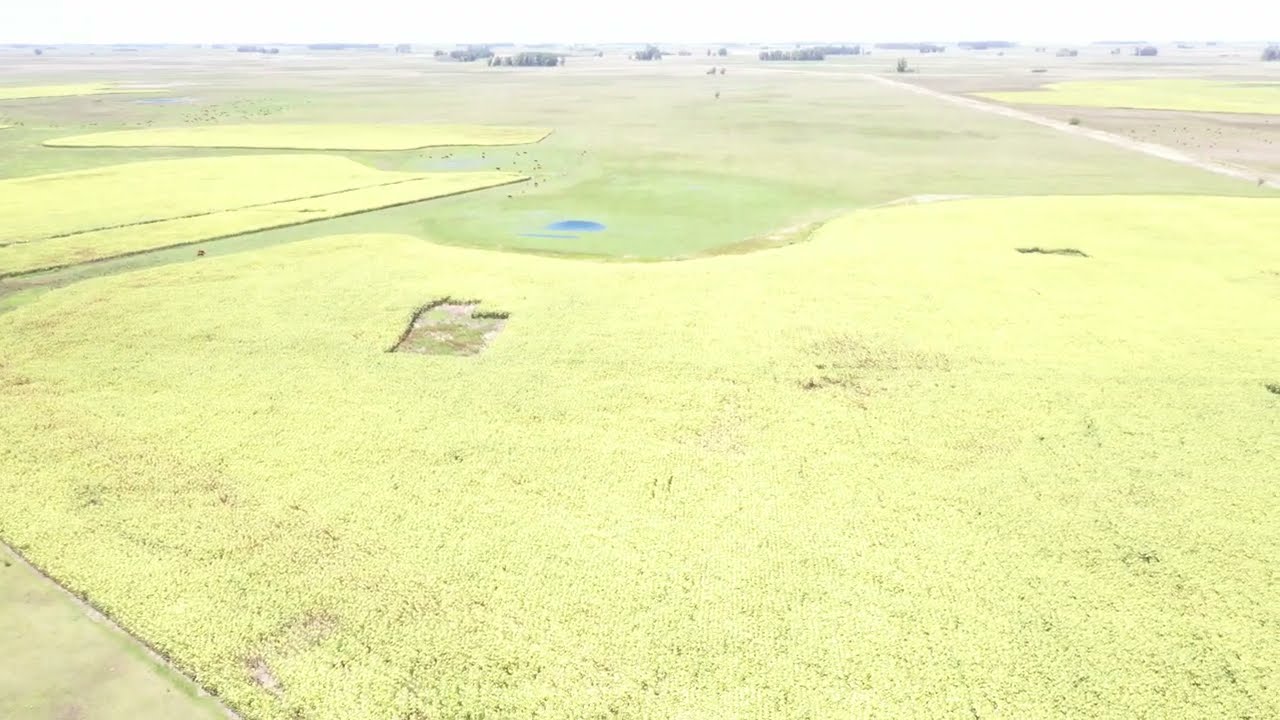This is an overhead, daytime photograph of a rural farm area featuring an overexposed, faded color palette dominated by shades of yellow, green, and brown. The center of the image showcases a blue pond nestled within a circular depression of greener ground. The fields, mostly a bright yellow hue due to the overexposure, spread out across the scene with a variety of agricultural patches. In the upper right-hand corner, a dirt road cuts diagonally from the lower right to the upper left. Towards the background, particularly at the top of the image, small groves of trees are faintly visible. The sky appears almost white, washed out by the intense light, further emphasizing the hazy, indistinct quality of the photograph. Below the pond and towards the left, there is a peculiar, leaf-shaped cut made into the yellowish plants, adding a curious detail to the otherwise expansive fields.